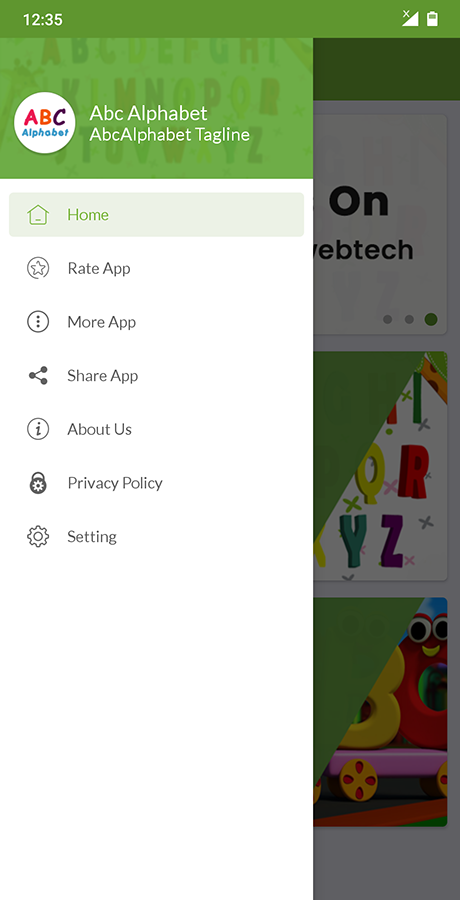This smartphone screenshot captures a detailed view of a green and white web page at 12:35. In the top-right corner, two icons are displayed—a battery icon and a Wi-Fi icon labeled "plus," with this section of the screen highlighted in green. The prominent green banner extends across the page. Below this banner, a white circle contains the text "ABC Alphabet," alongside a tagline "ABC Alphabet Tagline." 

The site features several vertical tabs on the left, each accompanied by illustrative icons:
- Home (house icon)
- Rate App (star icon)
- More App (three dots in a circle)
- Share App (sharing connection icon)
- Information (about us, indicated by an 'i' within a circle)
- Privacy Policy (lock icon)
- Settings (gear icon)

On the right side of the screen, there appears to be a dark overlay covering approximately a quarter of the page, partially obscuring the display. Visible text includes "O-N," and fragments "E-B-T-E," with three dots accompanied by the letters "I-Q-R-Y-Z." Additionally, children’s play blocks are present, possibly providing a playful design element to the web page.